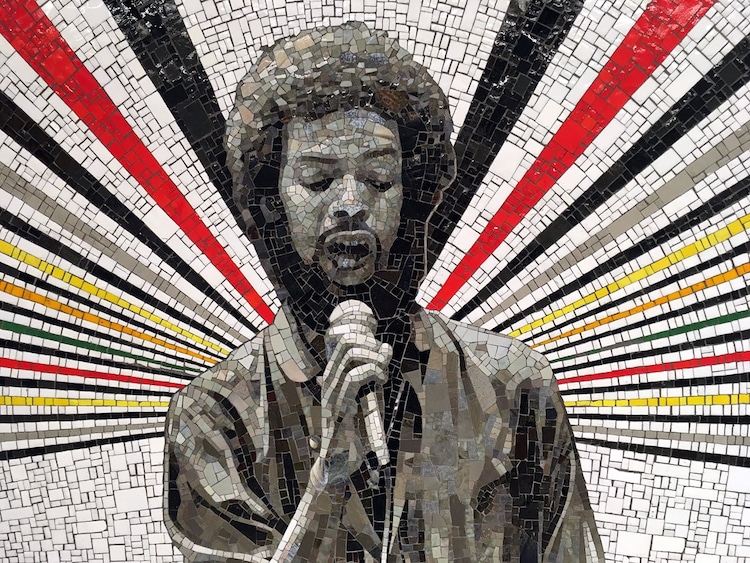The image showcases an extensive color mosaic artwork depicting a man, reminiscent of Jimi Hendrix, holding a microphone. Created using large squares of various solid colors and sizes, this mosaic assembles into a near photorealistic portrayal. The man, centrally positioned, has black curly afro hair and a large bushy beard with a goatee and mustache. His eyes are closed, and his mouth is open, as if passionately singing into the microphone held in his right hand. He is clad in a dark suit, which some interpret as brown, providing a stark contrast to the dynamic multicolored lines—featuring shades of red, black, yellow, orange, and green—that radiate outward from behind him against a white backdrop, suggesting an almost tunnel-like perspective. The artwork's vibrant tiles create an intricate and vivid scene, evoking the intensity and spirit of his performance.